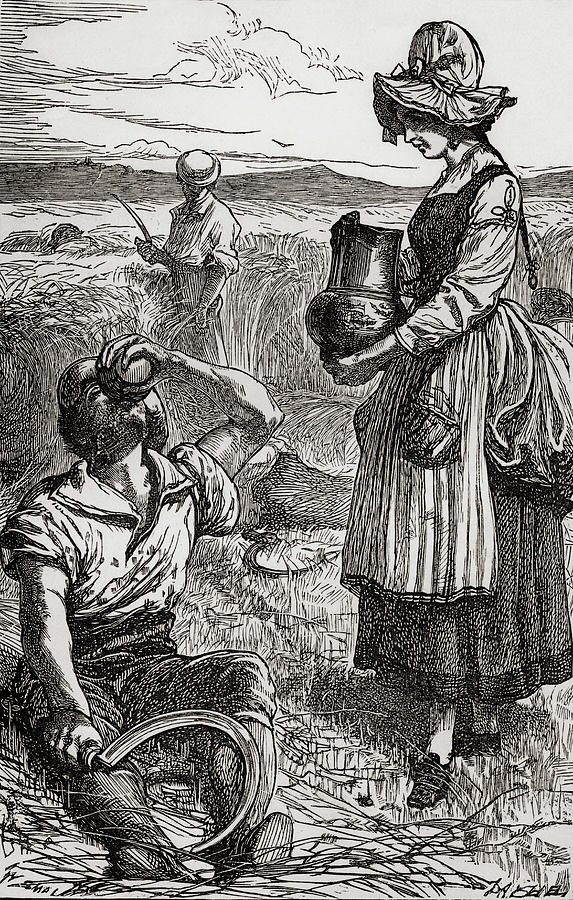This black-and-white drawing, likely set in the early 1900s in a European countryside, captures an evocative farming scene. In the foreground, a woman dressed in a long work maid's dress, complete with an apron and a wide-brimmed sun hat adorned with flowers, offers water from a pitcher to a man seated on the ground. The man, clad in a shirt, dark pants, boots, and a straw hat, is taking a drink from a cup in his left hand, while his right hand rests on a sickle lying across his knee. To their side, tall wheat or grass surrounds them, with another figure in the background. This second man, possibly another worker, stands upright with a sickle in hand, actively harvesting the crops. Behind them, detailed black-and-white clouds and a distant mountain range complete the pastoral scene, with an unreadable inscription at the bottom, likely the artist's signature.